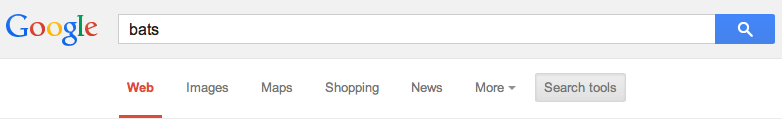This image is a screenshot of the Google search engine interface from several years ago, showcasing an older design that was in use at the time. At the top of the page, there is a light gray header featuring Google's old logo. The logo displays the letters in the traditional Google colors: blue 'G', red 'o', yellow 'o', blue 'g', green 'l', and red 'e', but in Google's former font style. 

The search box in the center of the page is square-shaped rather than the modern rounded design. To the far right of this box is a blue rectangle containing a white search icon. The search term entered in the box is "BATS" (spelled B-A-T-S). 

Below the search box, none of the search results are visible, but the navigation menu is clearly displayed as it appeared in that era. The "Web" option is highlighted in red with a red underline beneath it. To the right of this, in gray font, are other options: "Images," "Maps," "Shopping," "News," and "More," with the "More" option displaying an inverted triangle indicating a dropdown menu. To the far right is "Search tools" housed in a light gray rectangle with slightly darker gray font. This menu demonstrates the typical Google search interface elements users would have encountered a few years ago.